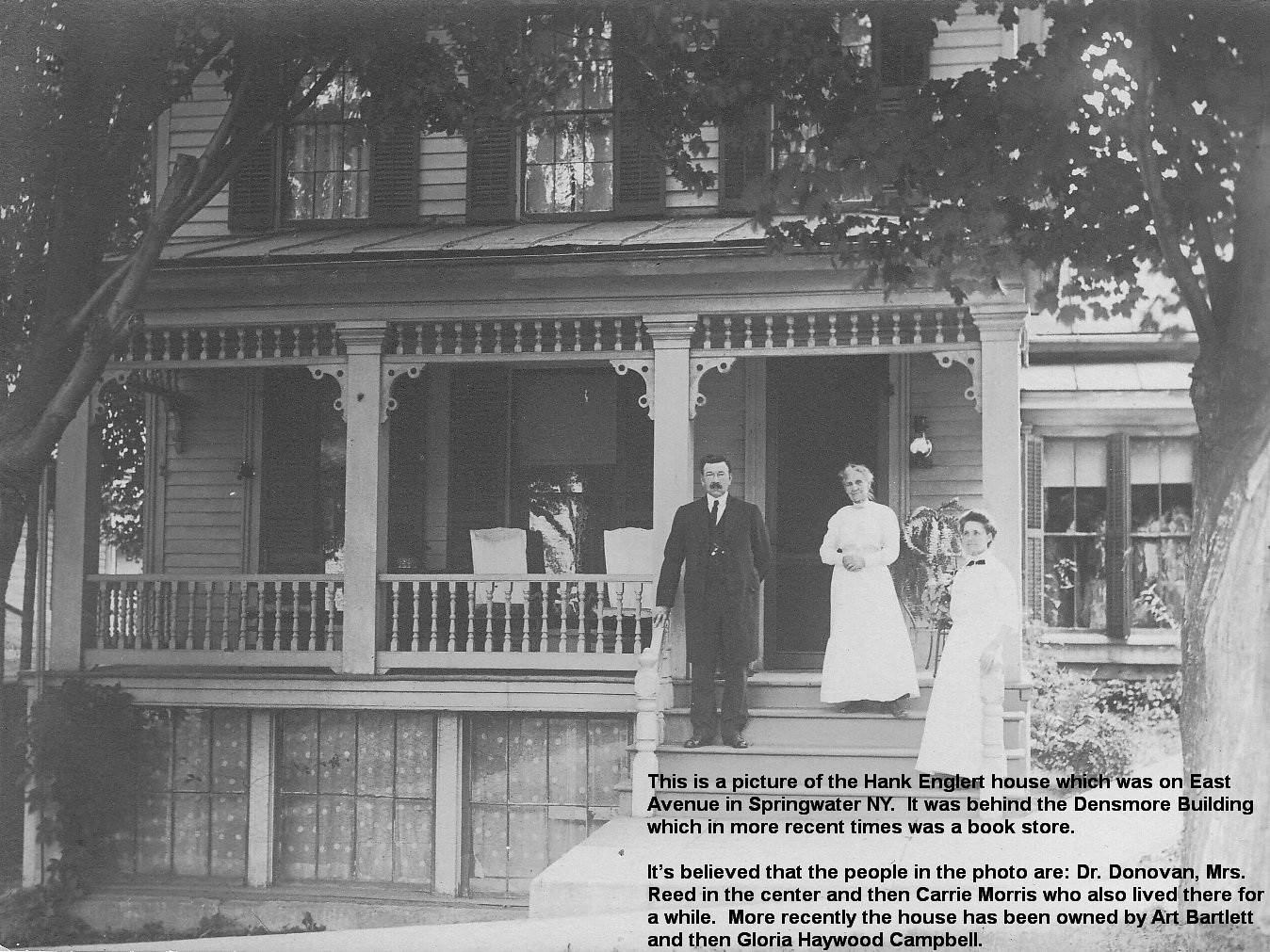The image features a historical black-and-white photograph of the Hank Engler House, located on East Avenue in Springwater, New York. Dominating the background is the facade of the house, which includes a long front porch with a staircase descending to the sidewalk at the center. Standing on the porch and facing the camera are three individuals: a gentleman in a three-piece suit identified as Dr. Donovan, a lady in a long white dress at the center, identified as Mrs. Reed, and another lady in a white dress with a black bow tie, identified as Carrie Morris. The text in the bottom right corner of the image confirms these details and notes that the house, recently owned by Art Bartlett and Gloria Haywood Campbell, was historically situated behind the Densmore Building, which was a bookstore in more recent times. The monochromatic hues of black, white, and various shades of gray suggest that the photograph was taken several decades ago.